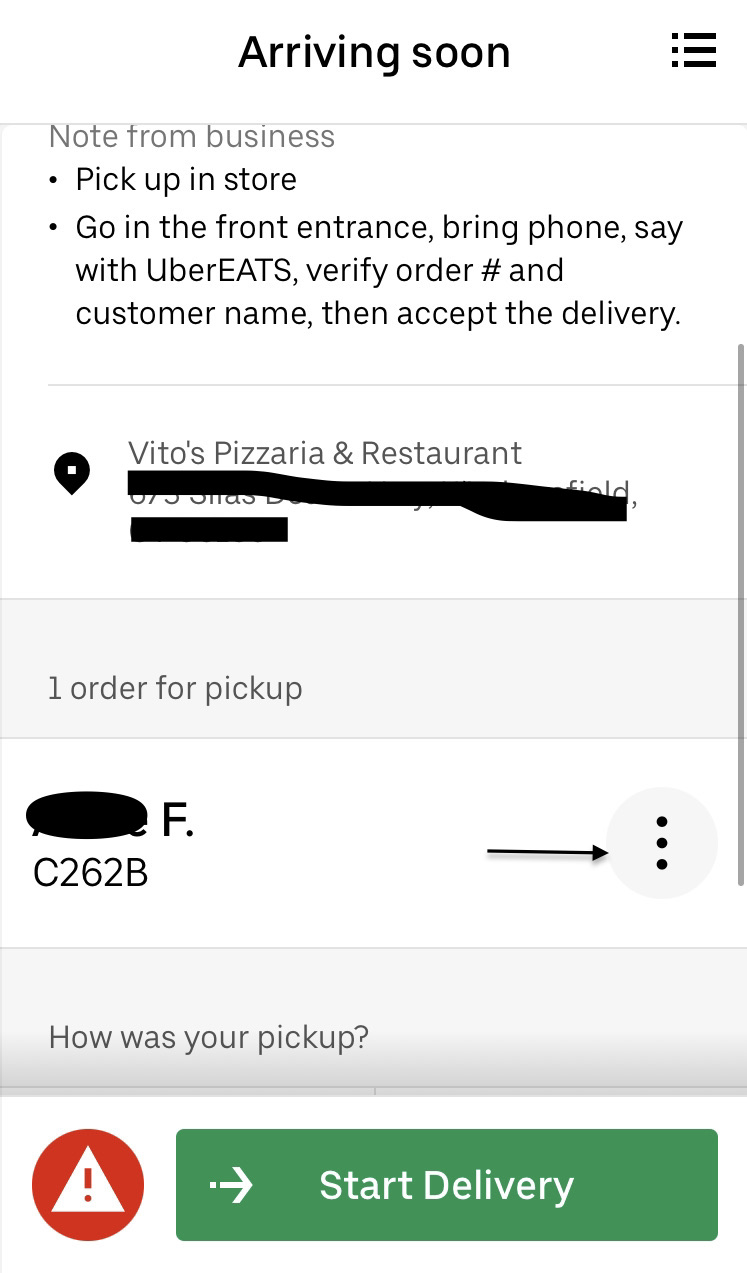The image is a vertically oriented mobile screenshot showcasing delivery information for an Uber Eats order. At the top of the screenshot, the text "Arriving Soon" is displayed prominently in black. In the top right-hand corner, there are three horizontal bars, each with a black dot to the left. The background of the image is entirely white, creating a clean and minimalistic look.

Beneath the top section, a gray text box labeled "Note from business" appears, followed by two bullet points. The first point instructs, "Pick up in store." The second point reads, "Go to the front entrance, bring phone, say with Uber Eats, verify order number and customer name, then accept the delivery."

Below these instructions, there is an address section for the restaurant, partially obscured. A black, upside-down teardrop-shaped icon with a white dot inside precedes the text "Vito's Pizzeria and Restaurant." Portions of the address have been redacted with a black marker for privacy.

Further down, a gray rectangle contains the text "1 order for pickup" in its bottom left-hand corner. Directly below, a white rectangle shows the customer's first name obscured by a black oval, revealing only the initial "F" of their last name. An alphanumeric code "C262B" is displayed beneath this.

To the right of the customer's name is an arrow pointing to three vertical dots. Underneath this section, the text "How was your pickup?" is displayed in gray. Finally, at the very bottom of the screen, there is a prominent green button labeled "Start Delivery."